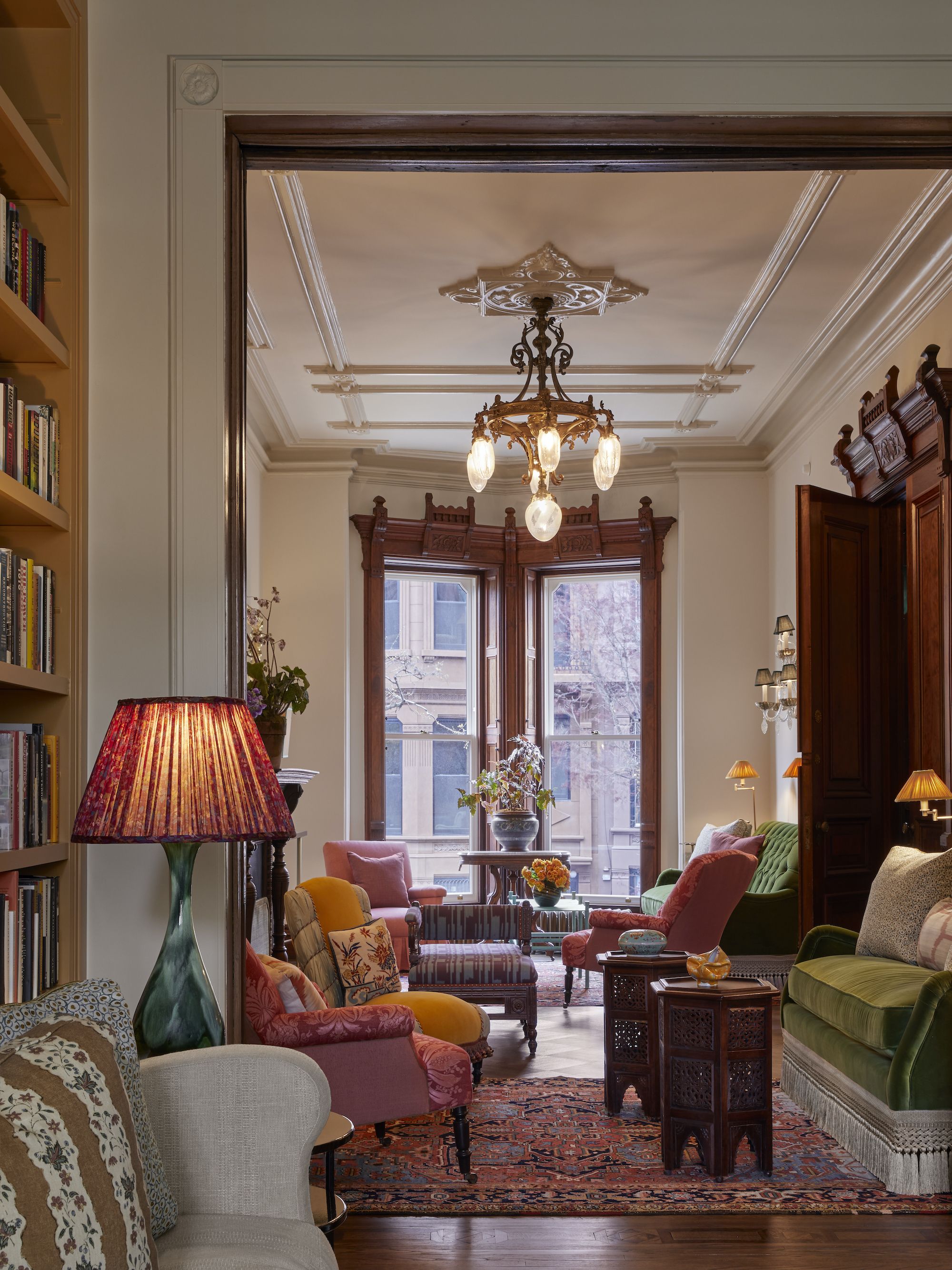This image captures the refined interior of a well-appointed living room or parlour within an elegant, possibly Victorian-era brownstone. The living space boasts impressively high ceilings, likely around 12-13 feet, adorned with intricate crown molding and a medallion centerpiece from which hangs an antique brass or bronze light fixture. The walls and ceilings are painted in a creamy hue, contributing to the room’s airy and sophisticated ambiance.

The floor-to-ceiling windows, trimmed in beautifully carved dark wood, allow a view of similar historic buildings across the urban street, hinting at the home’s brownstone neighborhood. Within the room, there is a mix of plush, green-upholstered furniture with white fringe trim, including a fancy green couch and matching love seat. The seating area is tastefully arranged with tan throw pillows and a few rose-colored chairs, complemented by intricately carved wooden tables. 

A green couch with tassels is visible just within the frame, hinting at another room or a secondary seating area visible through an open doorway. This room features a large bookshelf that stretches up the wall, indicating an impressive collection of books.

The space is richly decorated with ornate light fixtures that have a jade-like body and red shades, as well as an elegant oriental rug that delineates the seating arrangements. The entire scene is tied together by the luxurious elements and meticulous attention to detail, reflecting the opulence and timeless elegance of a bygone era.